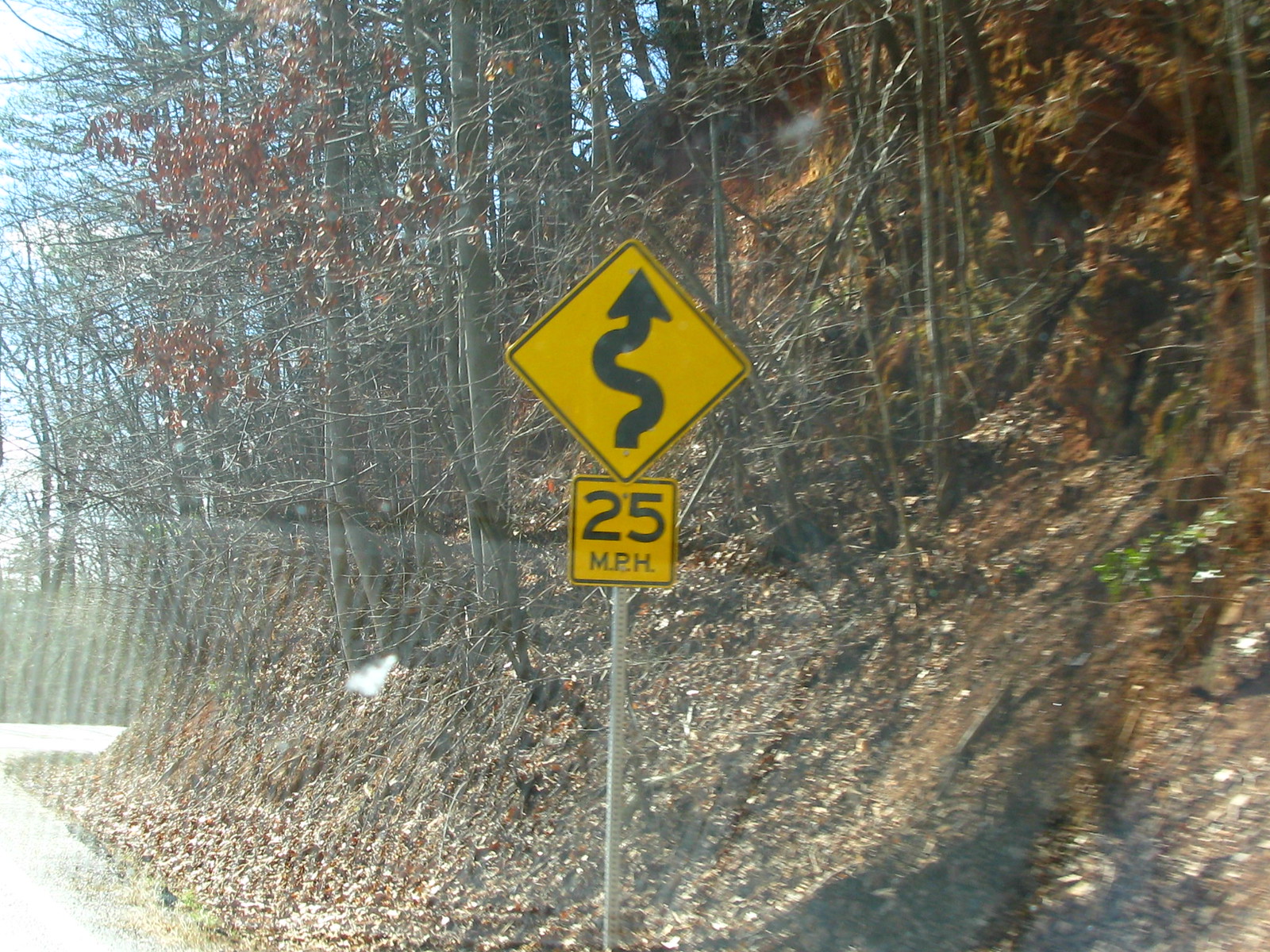The photograph depicts a road sign mounted on a gray pole. The sign consists of two parts: the upper part is a diamond-shaped, yellow sign bordered in black, featuring a winding arrow that curves right, then left, before pointing upwards, indicating a winding road ahead. Beneath this, there is a smaller, square yellow sign with a black border displaying "25 MPH," indicating the suggested speed limit. To the right of the sign, there is a steep hill densely populated with trees, many of which have shed their leaves, revealing a mix of brown and dark red foliage scattered among the bare branches.